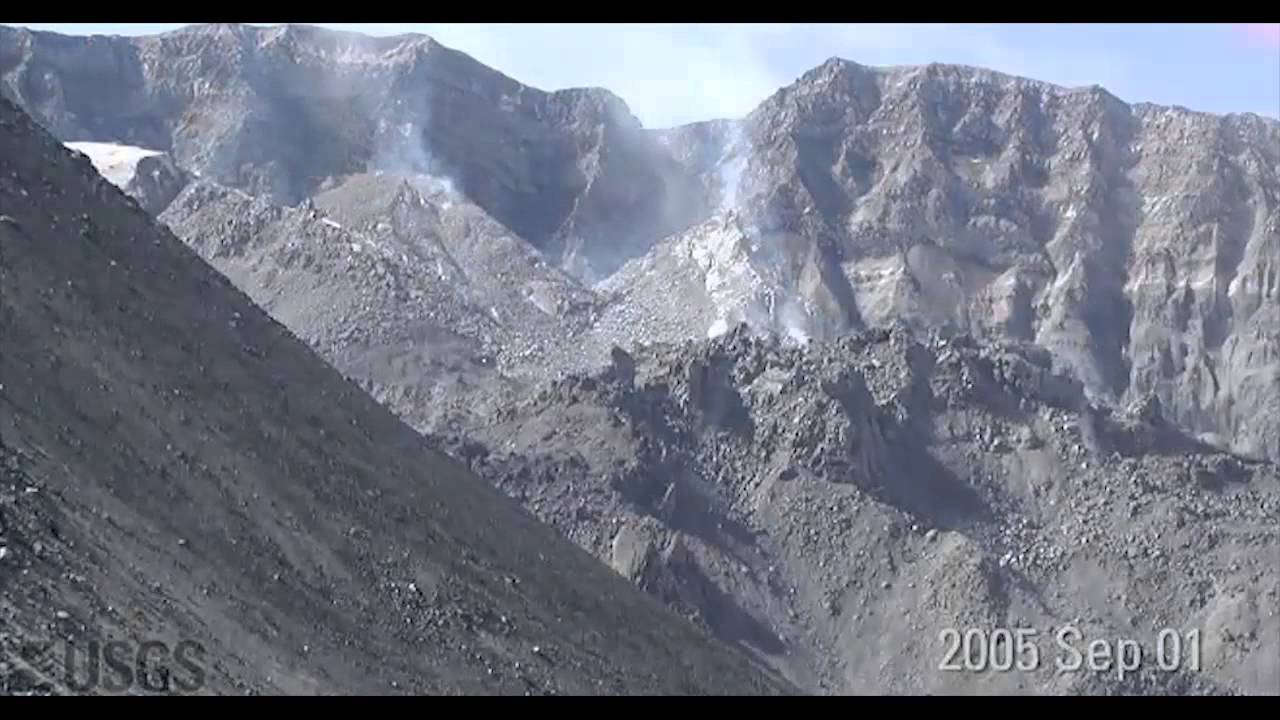The image appears to be a trail cam photograph, dated September 1, 2005, as indicated by the timestamp "2005 SEP01" in the bottom right corner. In the bottom left, the watermark "USGS" suggests it might be from the United States Geological Survey. The photograph captures a rugged, mountainous landscape. The scene is dominated by various shades of gray, highlighting the texture of the terrain. In the foreground, a steep, sloped part of the mountain is visible, composed of smaller, thinner rocks. Behind this, a ridge transitions to a hillier area. Further in the background, more defined rock formations are prominent, featuring large, distinct pieces. A faint trace of smoke can be seen rising from the mountainside. At the very top of the image, a sliver of blue sky is visible, adding a touch of color above the predominantly rocky and cliff-filled landscape. The sky is mostly clear with minimal cloud cover, and a bit of sunlight filters through, enhancing the stark contrasts within the frame.